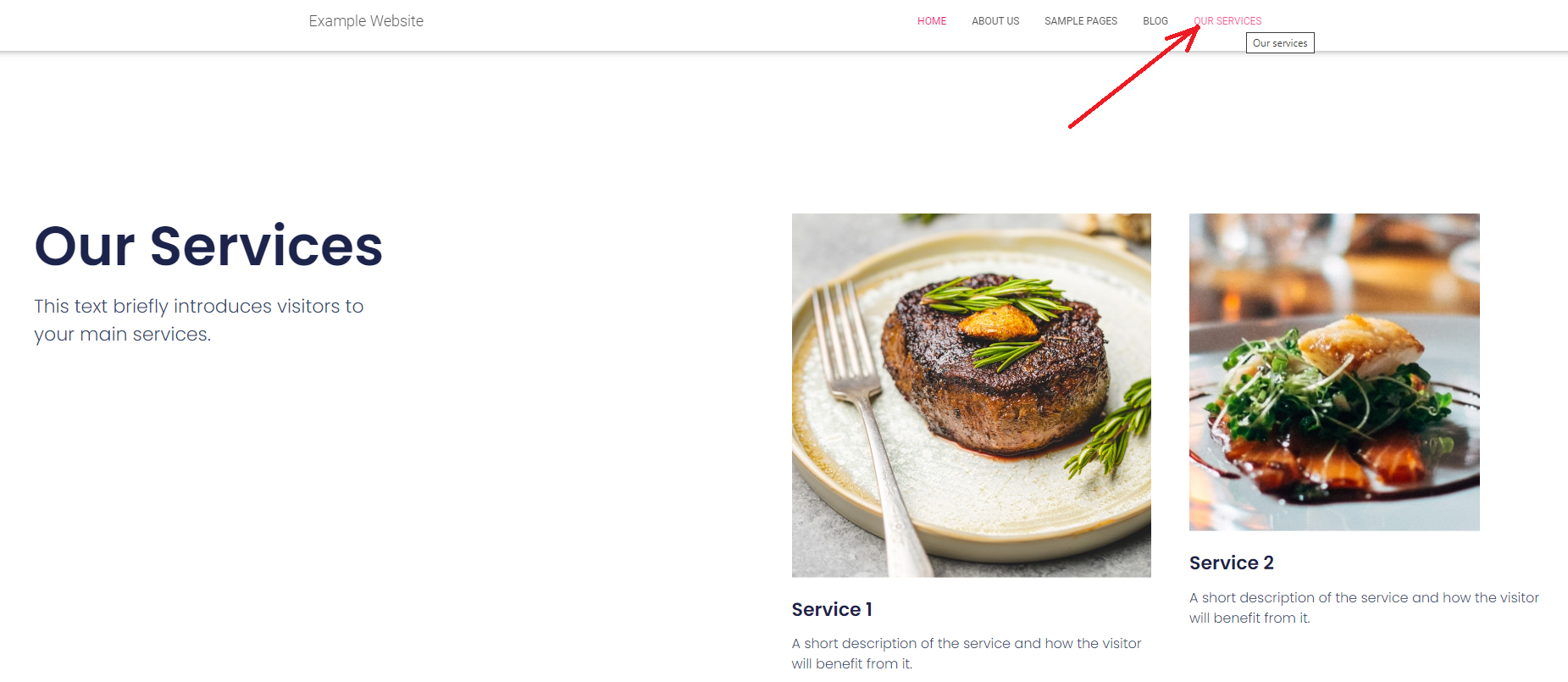This detailed screenshot showcases the homepage of an unidentified website. The top navigation bar features the following menu items: "Example Website," "Home," "About Us," "Sample Pages," "Blog," and "Our Services." A prominent red arrow points diagonally upwards towards the right, highlighting the "Our Services" section with emphasis specifically on the word "Our."

On the left side of the page, the heading "Our Services" is visible, accompanied by introductory text that briefly describes the primary services offered to visitors. To the right, there are two high-quality photographs that elaborate on the services visually.

The first photograph features a beautifully grilled steak with a caramelized crust. It is garnished with a small triangular piece of an unknown material, possibly an edible decoration, and some fresh leafy green herbs. This appetizing steak is presented on a rustic earthenware plate, with a silver fork positioned on the left side. Below this image, there is a caption that reads: "Service 1," followed by a brief description outlining the service and its benefits to the visitor.

The second photograph depicts an array of dark pieces of fish, generously covered in a rich, brown sauce. Garnished with microgreens and a rectangular brown item placed atop the microgreens, the dish is artfully drizzled with a dark brown sauce on the plate. Below this enticing image, the caption reads: "Service 2," accompanied by a concise description that details the service and its advantages for the visitor.

This screenshot not only captures the visual and textual elements of the webpage but also provides a detailed insight into the services offered, making it informative and visually engaging for the viewer.